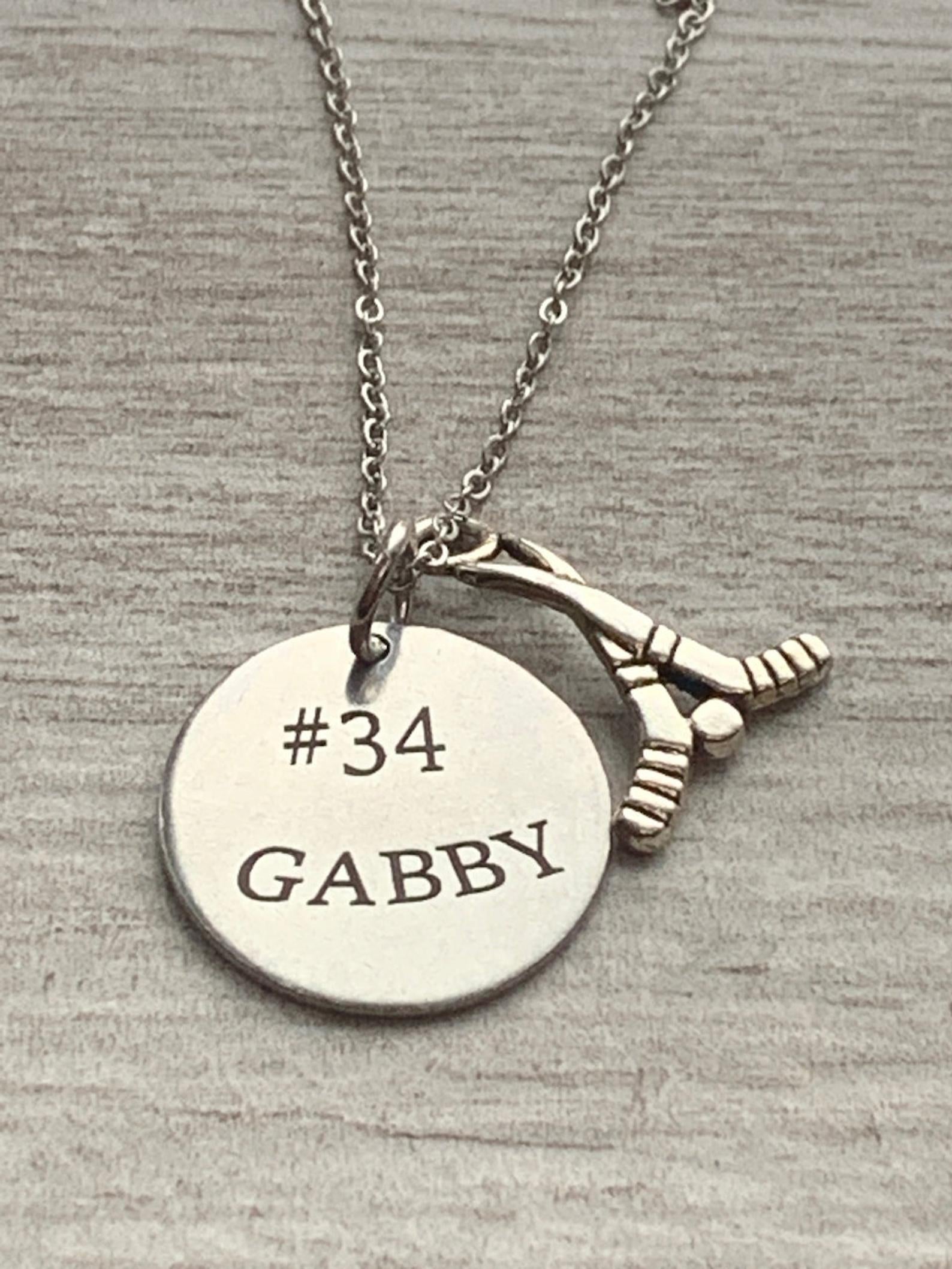The image features a delicate, light gray metallic necklace with a small chain link design, exhibiting a shiny, steel-like appearance. The necklace includes a central clasp connecting two distinct pendants. The primary pendant, connected directly to the clasp, is a thin, circular piece of metal with an engraving that reads "Number 34, Gabby". To the right, another pendant depicts two crisscrossed hockey sticks, also metallic, with a small puck situated at their crossing point. The entire ensemble is laid out against a beige or grayish fabric background, enhancing the necklace's metallic sheen.